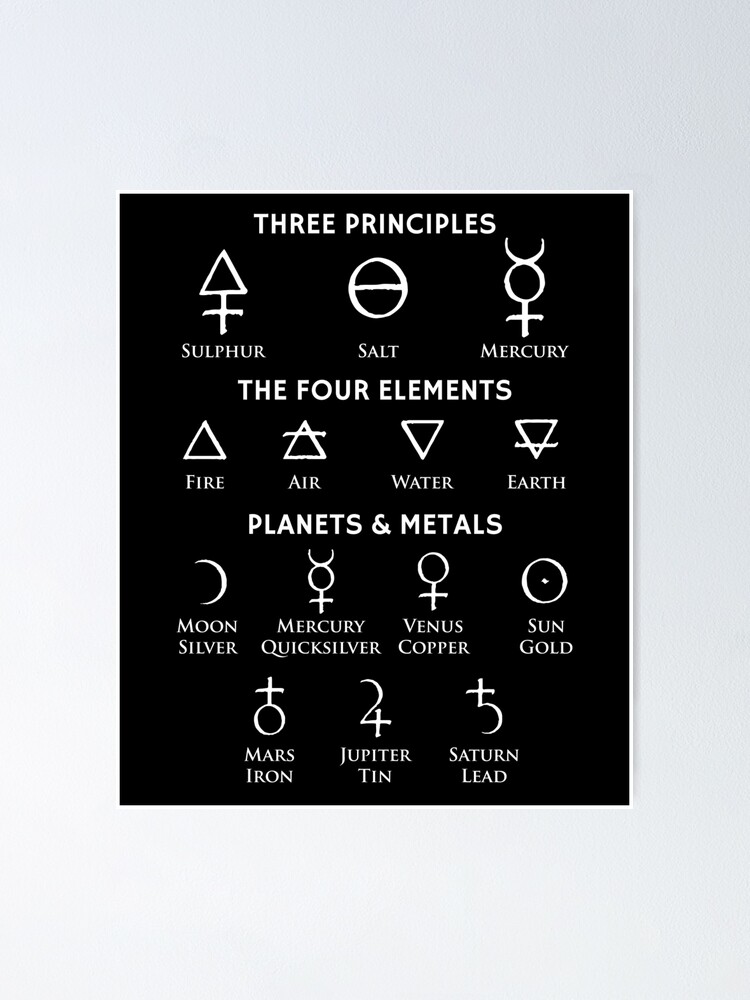The image features a detailed diagram set against a simulated white wall background, resembling a poster with a thin white border around it. The central portion of the poster has a black background with white text and intricate symbols. At the top, in bold capital letters, it declares, "THREE PRINCIPLES," followed by their corresponding alchemical symbols: sulfur (an upward arrow with a horizontal line), salt (a circle with a horizontal line), and mercury (a circle with a cross below and a 'U' shape on top). Below this, the poster lists "FOUR ELEMENTS," each represented by different triangle configurations: fire, air, water, and earth. The bottom section of the poster is titled "PLANETS AND METALS," which pairs celestial bodies with specific metals: Moon with silver, Mercury with quicksilver, Venus with copper, Sun with gold, Mars with iron, Jupiter with tin, and Saturn with lead, featuring their respective astrological symbols. The whole arrangement meticulously conveys alchemical associations through text and imagery.